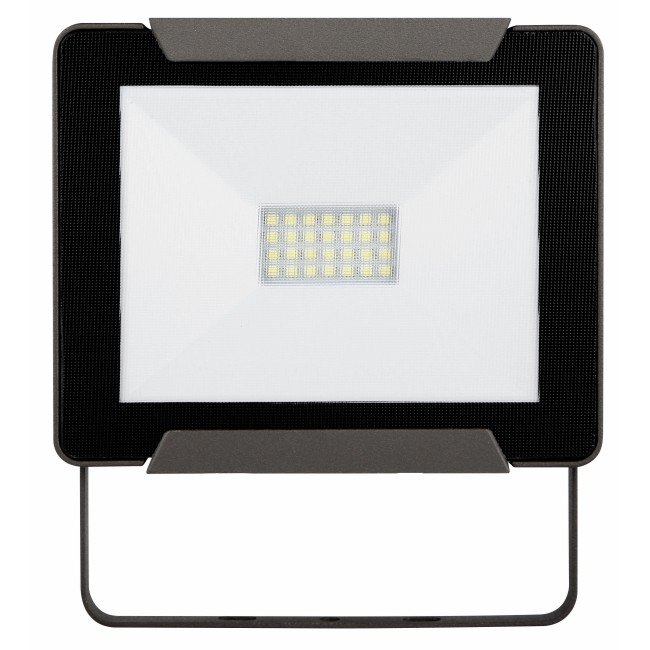The image depicts an up-close view of a tablet-like device with a thick black rectangular border approximately an inch wide. The screen within this border is predominantly white, featuring a grid pattern in the very center. This intricate grid comprises seven columns and four rows of squares, characterized by varying shades of green, including lime green, all framed by a darker green border outlining each square. The layout gives the impression of a pixelated image or a digital drawing. Additionally, the device has sturdy gray handles situated along the top and bottom of the screen, providing solid gripping points. Below the screen, a slender support structure, potentially made of metal or plastic, extends downward, suggesting it functions as a stand to keep the device upright, allowing it to be placed on a flat surface for display or use.